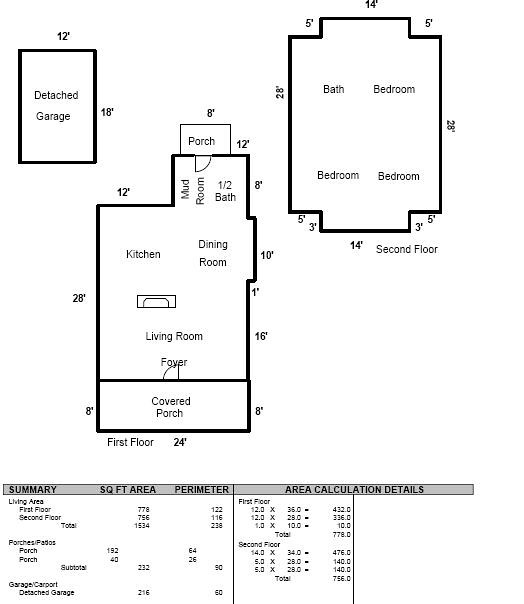This detailed image displays three distinct block layout plans, presumably of a multi-level home. 

The first layout, labeled as the "First Level," features a simple, blank square indicating a "Detached Garage" with dimensions of 12 by 18. 

The second layout, representing the main floor, is a square with a slight protrusion at the top. It details various rooms including a covered porch, foyer, living room, kitchen, dining room, mudroom, half bath, and another porch. 

The third layout, possibly the upper floor, is a square with indentations at the top and bottom. It identifies areas designated as bathrooms and three bedrooms. 

All three diagrams consist of basic outline drawings with textual placeholders noting the intended use of each space. None of the plans show interior walls, emphasizing the general layout rather than specific architectural details. Below the layouts, the image includes a summary providing square footage, perimeter, and area calculations, accompanied by additional information on these measurements.